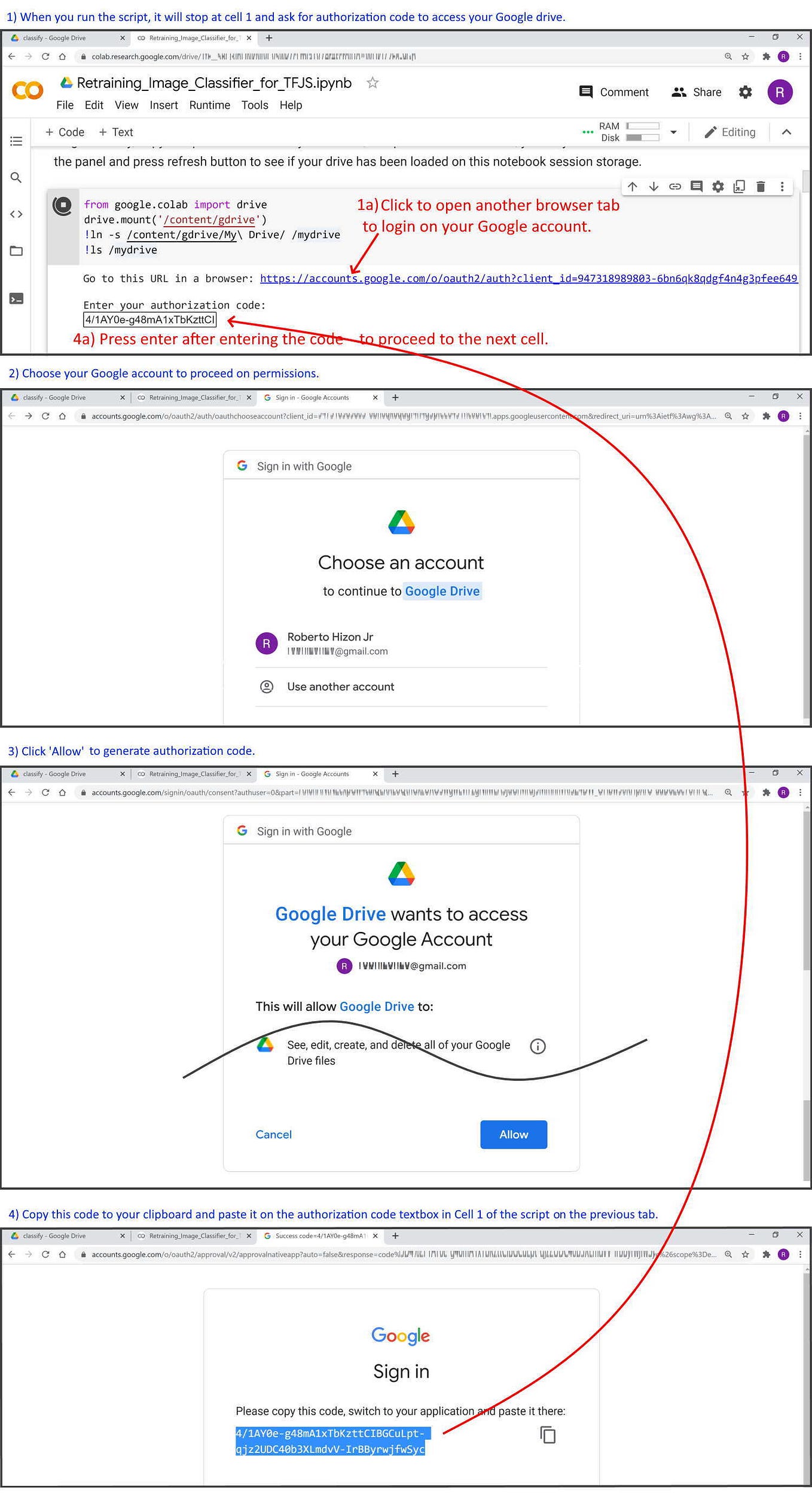**Caption:**

A collage featuring a tutorial on retraining an image classifier using TensorFlow.js. The sequence comprises four vertically aligned screenshots.

1. **Top Image:** The header text reads "Retraining Image Classifier for tf_js". The slightly overlapping circles representing a part of the TensorFlow.js logo are faint. 

2. **Second Image:** A profile icon in the upper right, a purple circle labeled "R", stands out. Two windows display a step-by-step guide.

3. **Directions Step 1:** The first screenshot indicates that running the script will pause at "call one" and request an authorization code to access Google Drive.

4. **Directions Step 2:** The second screenshot asks the user to choose their Google account.

5. **Directions Step 3:** The third screenshot instructs to click "Allow" to generate the authorization code.

6. **Directions Step 4:** The final screenshot guides the user to copy the generated authorization code and paste it into the specified text box in the script.

Each step is clearly labeled from one to four, showcasing the detailed instructions needed to complete the process.